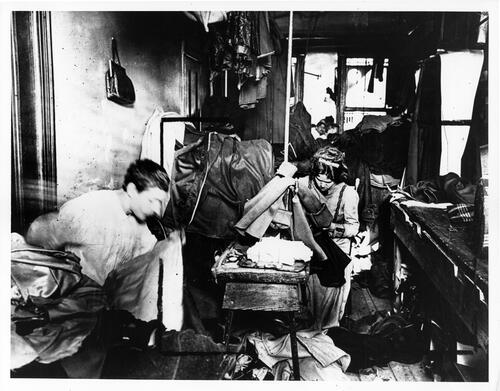This black and white photograph, likely taken in the 1940s or 50s, captures a bustling industrial setting, possibly a seamstress shop or makeshift clinic. The high-contrast image reveals a cluttered room filled with garments, bags, and various fabrics scattered throughout. In the foreground, a man with short brown hair, dressed in a white shirt, is crouched on the ground, engrossed in his work. To his right, a woman with puffy, short brown hair, also wearing a white garment, is bent over a table or suitcase, handling white clothes spilling out. The background features a wall lined with windows and more scattered items, contributing to the overall chaotic atmosphere of the space. The blur in the women's movements suggests they are caught in the midst of their tasks, highlighting the industrious and hectic nature of the scene.